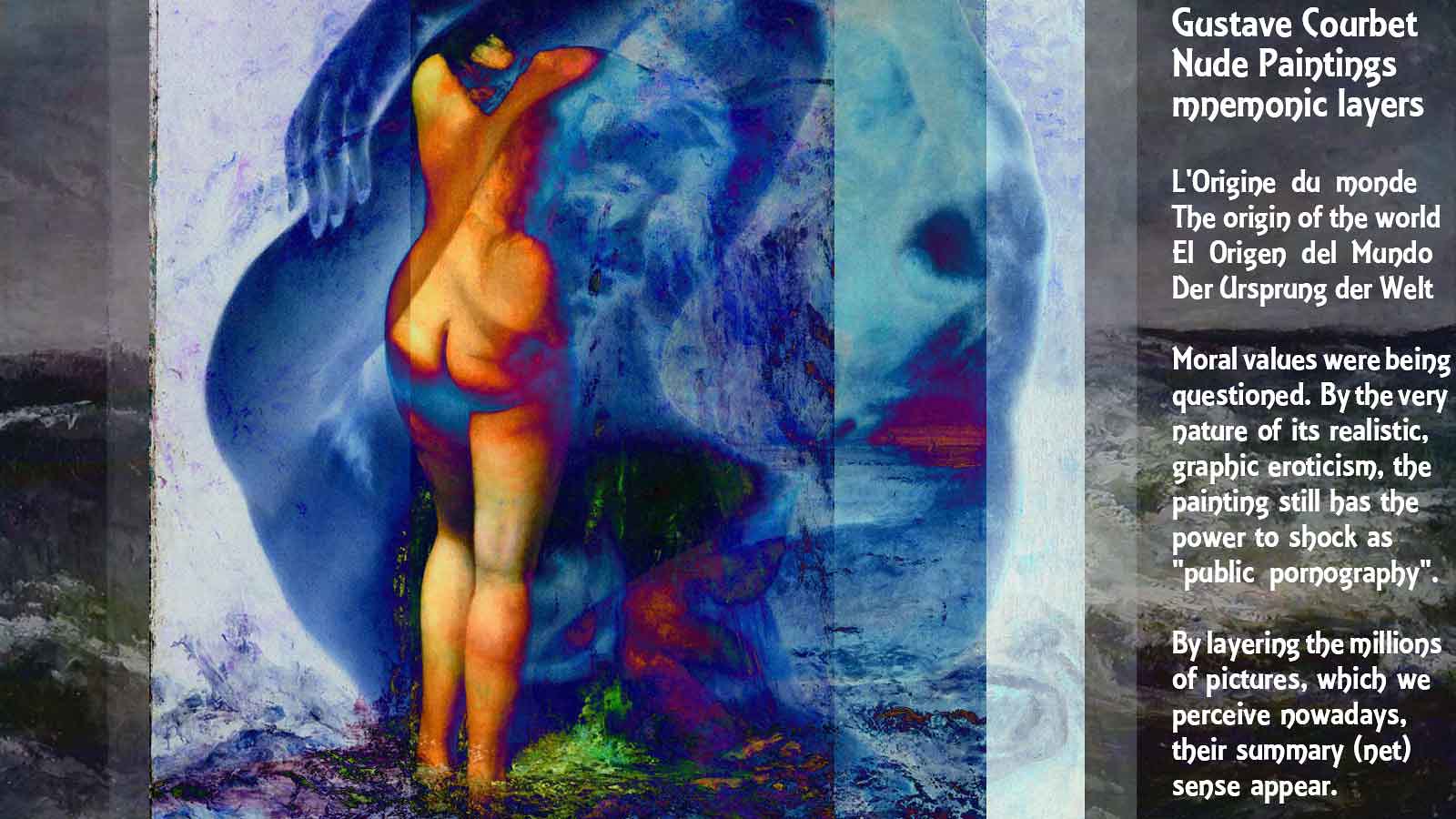The image is a detailed magazine article about the artist Gustave Courbet and his controversial nude paintings, prominently featuring one of his works titled "L'Origine du Monde" (The Origin of the World). The central painting depicts a nude woman standing with her back to the viewer, her arms raised above her head and her gaze directed downward. The abstract background of the painting is rendered in various shades of blue, with splashes of red, green, and black dispersed throughout.

In the foreground, within the blue hues, the woman's chest is clearly visible, including her right and left breasts and nipples. A blue shadow is noticeable beneath her buttocks, with green water splashing up from below. The piece is mounted on a gray marble surface.

On the right side of the image, there is text in multiple languages, including Spanish, Portuguese, English, French, and German. The text highlights the themes of Courbet's work, discussing how the realistic and graphic eroticism of his paintings continue to challenge moral values and provoke shock as public pornography. Phrases like "Moral values were being questioned" and "The painting still has the power to shock" emphasize the enduring impact of Courbet's art. The titles in different languages reinforce the universal recognition of the piece.